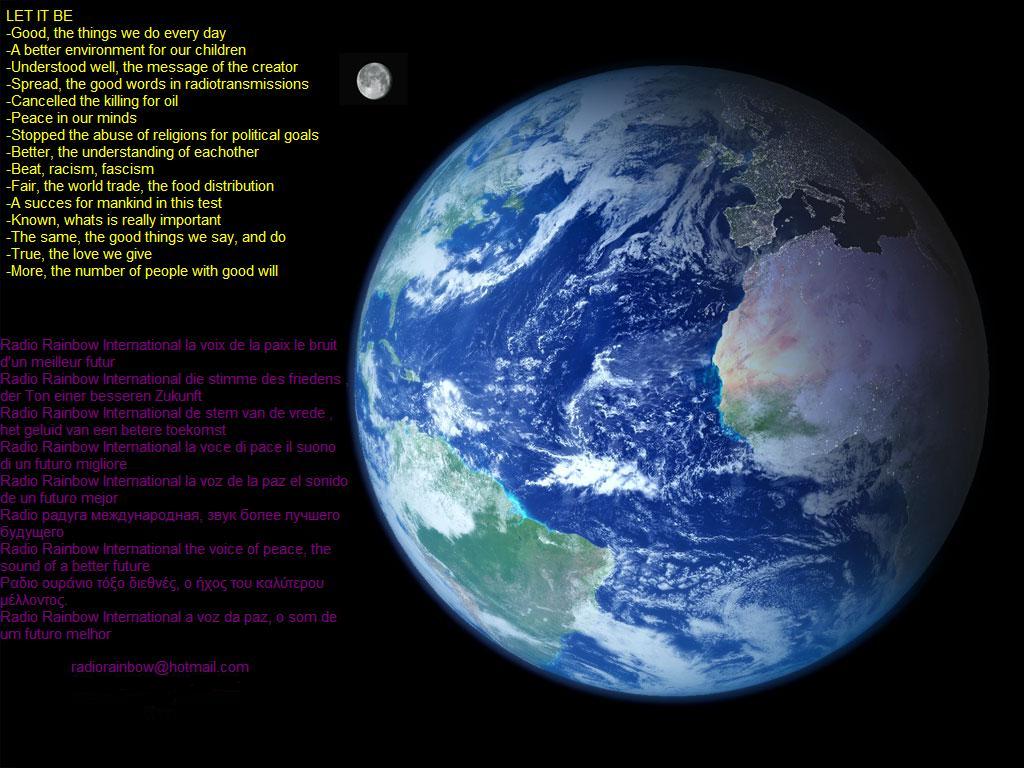The image showcases a striking view of Earth from space, set against a deep black background. Dominating the right-hand side of the image, the Earth reveals parts of North America, South America, a significant portion of Africa, most of Europe, and some of the Middle East and Asia, all framed by vast expanses of ocean dotted with wispy clouds. Nearby, the moon appears as a small round circle toward the top right. On the left-hand side, the image features detailed text sections. At the top, in bold yellow capital letters, are the words "LET IT BE," followed by 15 lines of thought-provoking bullet points that advocate for peace, environmental care, understanding, and global goodwill. Below this, another section of text in purple discusses similar themes in multiple languages, although the readability is somewhat compromised due to JPEG compression. Centered beneath the purple text is an email address: RadioRainbow@hotmail.com.